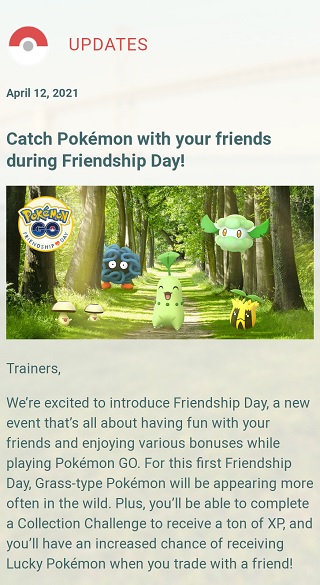The screenshot displays an update from the Pokémon GO app, featuring a Pokéball symbol at the top alongside the word "Updates" in red font. The update is dated April 12, 2021, and is presented in an article-like format. The headline reads, "Catch Pokémon with your friends during Friendship Day," followed by a banner image showing several Pokémon in a forest setting, accompanied by the Pokémon GO Friendship Day logo, positioned in a circle on the left side. 

Below the image, the notice begins with "Trainers," introducing Friendship Day—a new event focused on enjoying the game with friends and benefiting from various in-game bonuses. The notice explains that during this initial Friendship Day event, grass-type Pokémon will appear more frequently in the wild. Players can also complete a collection challenge to earn significant XP and will have an increased likelihood of obtaining lucky Pokémon when trading with friends. This completes the update, which serves to inform players of the upcoming seasonal changes and events in the game.